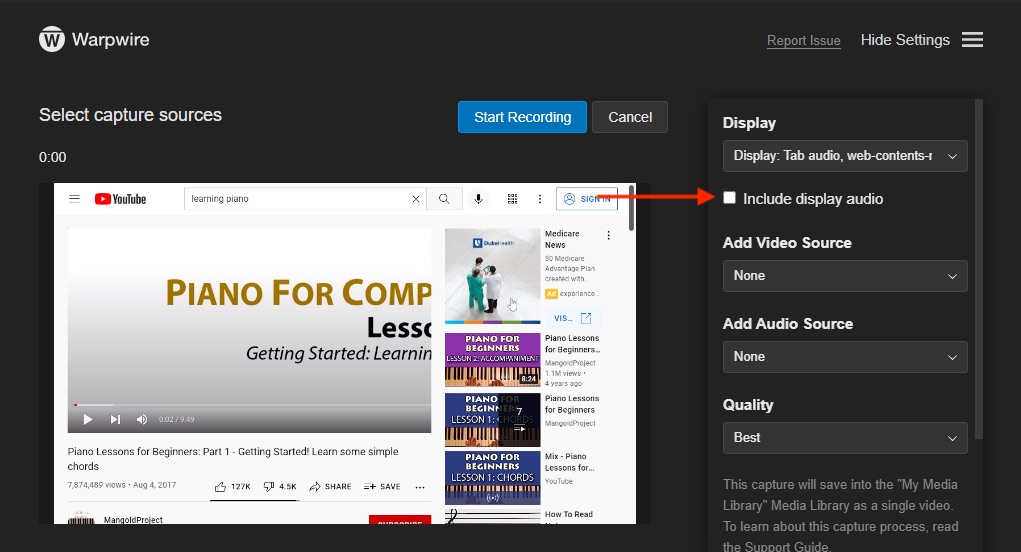The website interface in the image is called Warpwire, with the name "Warpwire" clearly displayed in the top-left corner. On the top-right corner of the screen are options labeled "Report issue," "Hide settings," and a menu icon represented by three horizontal lines stacked on top of each other. 

On the left side of the interface, there's a section titled "Select capture source," followed by a prominent blue button labeled "Start Recording" in white font. Next to this is a black button labeled "Cancel" in white font. Below these buttons, the interface resembles a YouTube page featuring a video titled "Piano for COM." There is also a "Sign In" button, accompanied by a red arrow pointing towards the "Include display audio" option on the right side of the screen.

On the right side, a list of options is visible:
- "Display"
- "Display Tab"
- "Audio"
- "Web Content" with a dropdown menu

Below these options is a checkbox labeled "Include display audio," which is highlighted by the aforementioned red arrow, suggesting it is a key feature to be selected. Continuing downward, there is a prompt to "Add Video Source" with a dropdown menu currently set to "None." Immediately below, there is another prompt to "Add Audio Source," also set to "None" via a dropdown menu. The quality setting is indicated as "Best" with a corresponding dropdown menu for potential changes.

Finally, the interface explains that "This capture will save the info to 'My Media Library' as a single video," described within a frame at the bottom of the panel.